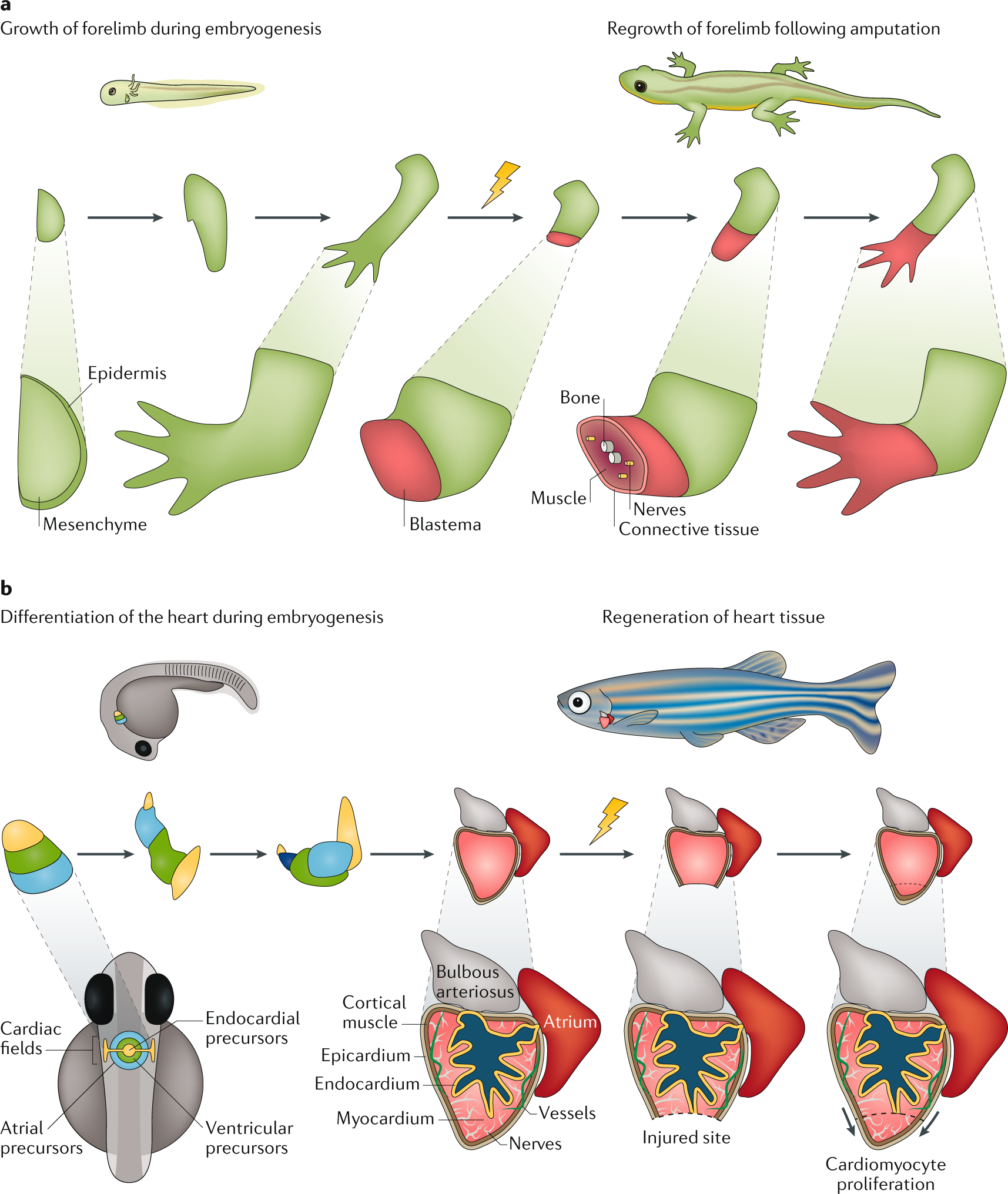This is a detailed color scientific illustration presented on a white background, divided into two main sections labeled 'A' and 'B'. 

Section 'A' is a diagram showing the "Growth of Forelimb During Embryogenesis" and "Regrowth of Forelimb Following Amputation" in an amphibian, specifically a salamander. The process is depicted through a series of stages, illustrated in pale green, red, and green, moving from a tadpole-like form to a fully grown salamander. Detailed captions identify the key stages of regeneration, including the reconstruction of bone, muscle, nerves, and connective tissue with arrows pointing to each part. 

Section 'B', located in the bottom half, focuses on a fish, depicting the "Differentiation of the Heart During Embryogenesis" and "Regeneration of Heart Tissue". The illustrations show the fish in grey with blue stripes and highlight the heart tissue in shades of red, blue, and slightly pinkish. This section includes flow chart-like diagrams with captions detailing the stages of heart tissue regeneration.

Each section includes call-outs to various anatomical parts and is adorned with a color-coded, cartoonized 2D drawing style for clarity. The overall layout resembles a scientific chart or poster typically found in biology textbooks.